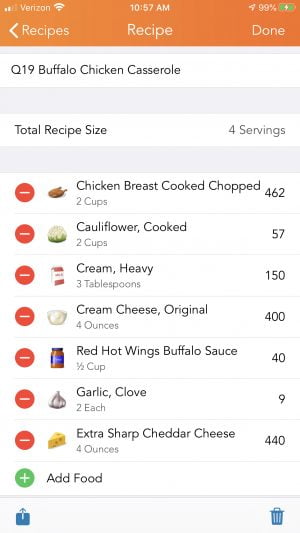This screenshot, captured from a cell phone, showcases a variety of interface elements. At the top, the banner is entirely orange, featuring white text that reads "Verizon." Adjacent to it, on the left, are the Wi-Fi signal indicator and the cellular signal bars. Centrally positioned is the current time, while the right-hand side displays the battery percentage. Below this banner, a secondary navigation header is visible in white text, stating "Recipes" on the left, "Recipe Done" in the middle, and a leftward-pointing arrow.

Underneath this header, there is a gray separator bar, followed by a white section. In bold black text within this white space, "Buffalo Chicken Casserole, Q19" is written. Below the title, another gray separator is present, followed by a white section that reads "Total Recipe Size for Servings."

Further down, another gray space separates the sections, leading into a list of ingredients organized by an icon system. The first ingredient, "chicken breast," features a stop sign icon to the left. Overall, the ingredient list includes items such as chicken breast and cauliflower, indicated as added items. Red buttons next to each ingredient suggest an option to remove them from the list.